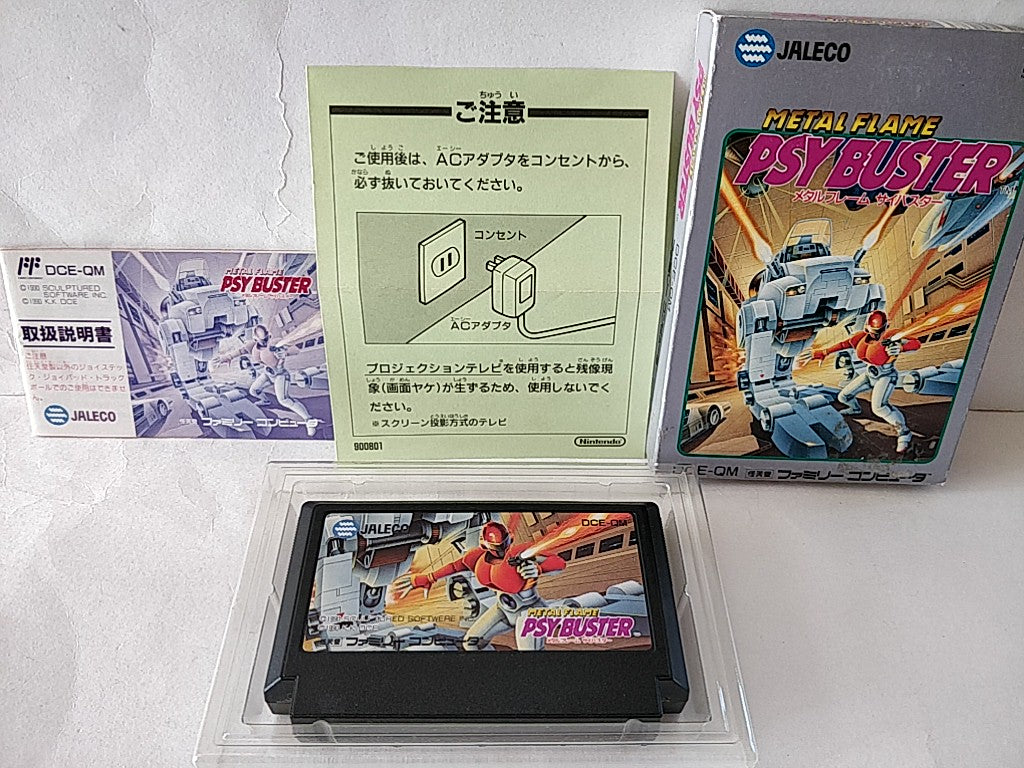The image is a detailed photograph, taken in full color with a horizontal orientation. It prominently features several items related to an old-fashioned video game. In the foreground, there's a clear plastic-encased black game cartridge for the game titled "Metal Flame Psybuster." The game box itself is also visible, displaying the title "Metal Flame Psybuster" in pink letters. The box art showcases a science fiction scene where a robot fires two cannons into the distance. In front of the robot, a character dressed in an orange helmet, an orange uniform, and white pants is also firing a weapon. The background of the box art includes a street with visible cars. The photograph also depicts two pieces of paper with instructions written in an Asian language, possibly Chinese or Japanese. One of the papers, which is green, includes an image of an electrical outlet with a plug plugged into it. These papers likely form part of the game manual, explaining how to use the cartridge and play the game.